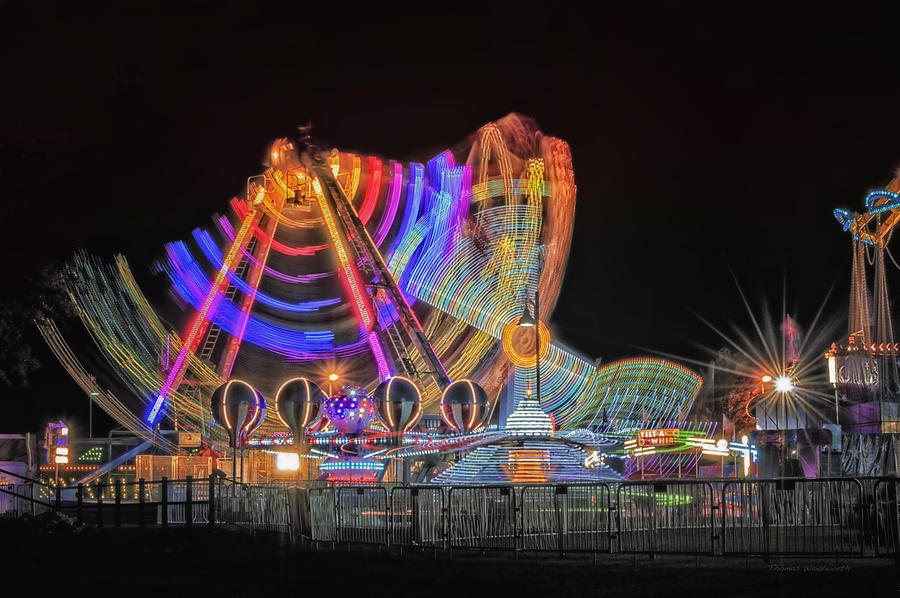This image captures a mesmerizing nighttime outdoor scene of a fair or carnival, set against an inky black sky and a shadowy foreground. A wrought iron fence, silhouetted and nearly blending into the darkness, spans the front of the fair, providing a stark contrast to the vibrant illumination beyond. Dominating the left side of the frame, a large ferris wheel radiates with motion-blurred neon colors of blue, orange, red, and yellow, creating a semi-circular arc of light. Below the ferris wheel, a row of whimsical, brightly lit hot air balloon structures adds to the kaleidoscope of glowing hues. To the right, additional rides, possibly a spinning attraction bathed in a bluish glow, along with other faintly discernible fair structures, emerge from the obscurity. The absence of people in the scene suggests an early setup or a prelude to the bustling activity typical of such fairs, further accentuated by the long exposure that blurs the dazzling lights into surreal streaks and shapes.